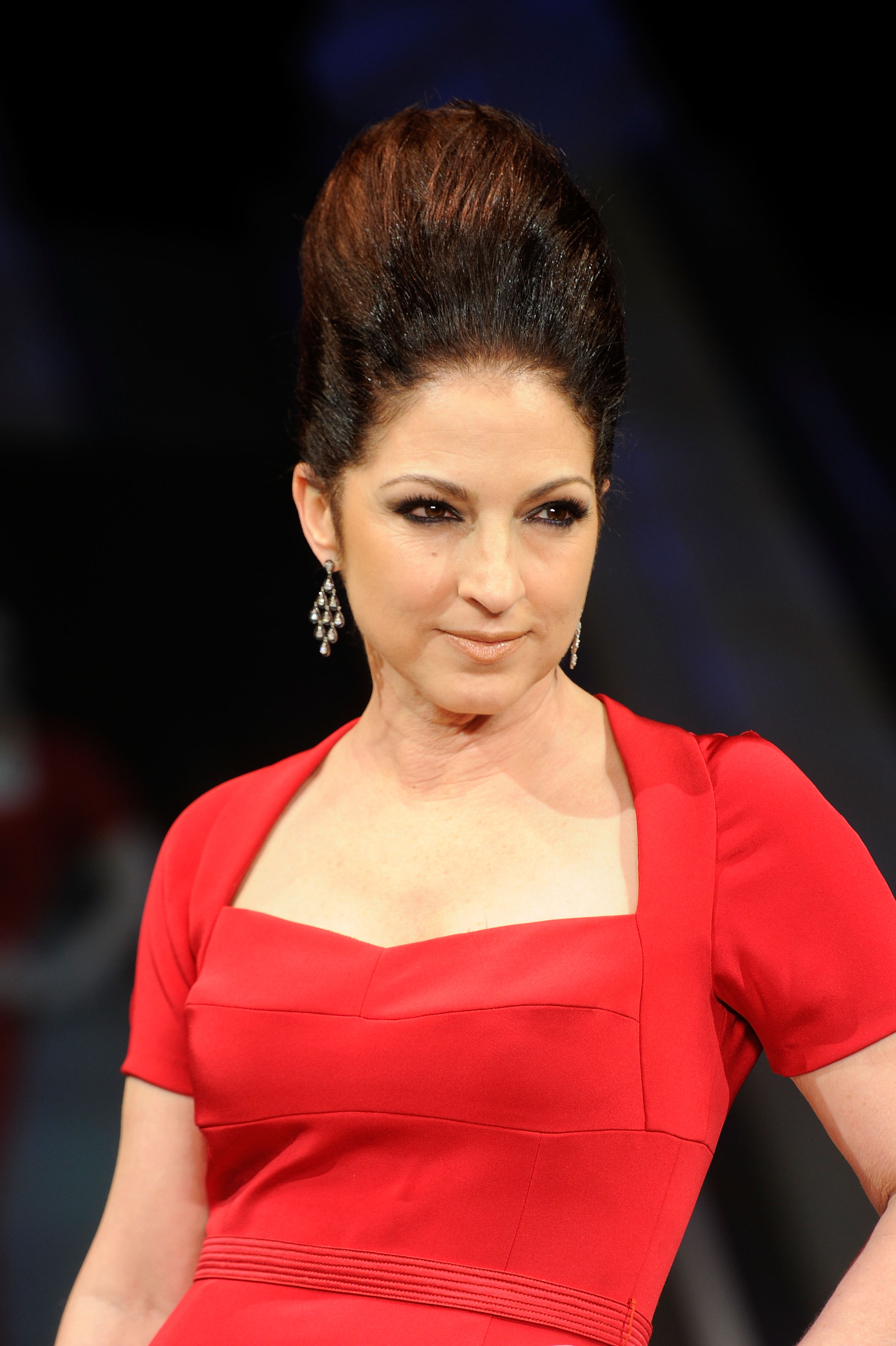The image is a vertically aligned rectangular photograph of a woman, viewed from the waist up. She is the sole subject in the photograph. She is dressed in a vibrant red dress with a square neckline and short sleeves, accentuating her elegant posture. Her hair is styled in an upward coiffure that resembles a beehive, blending shades of black and dark brown, with a hint of red at the back. She has a pair of diamond-shaped silver earrings, and her ears are clearly visible, not obscured by her hairstyle. 

Her body faces the camera, but she gazes intently off to the right, her face displaying a sense of intrigue. Her makeup is striking, with heavily penciled eyebrows and bold eyeliner highlighting her brown eyes. Although her left arm appears to be angled with a hand possibly on her hip, both arms are visible down to her waist. The background is indistinct due to the focus and lighting, merging into a blur of dark hues, which isolates and emphasizes her against a backdrop that appears to be black or dark shades of gray and brown. The overall composition draws attention to her poised demeanor and the detailed features of her appearance.